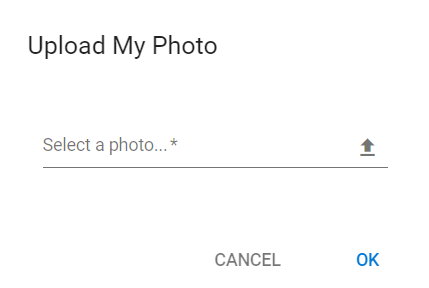The screenshot features a minimalist user interface layout on a completely white background. At the top, bolded text reads "Upload My Photo." Below this, a horizontal black line stretches across the screen with the prompt "Select a photo..." appearing above it, ending in an ellipsis that is accentuated by a star symbol atop the final dot. On the far end of this black line, a black upward-pointing arrow is positioned, indicating the button to click for uploading a photo. Beneath the black line, the word "Cancel" is displayed in standard text, with "OK" in blue letters positioned to its right. There are no additional images, colors, or background elements in the screenshot, maintaining a clean and straightforward design focused solely on the photo upload function.